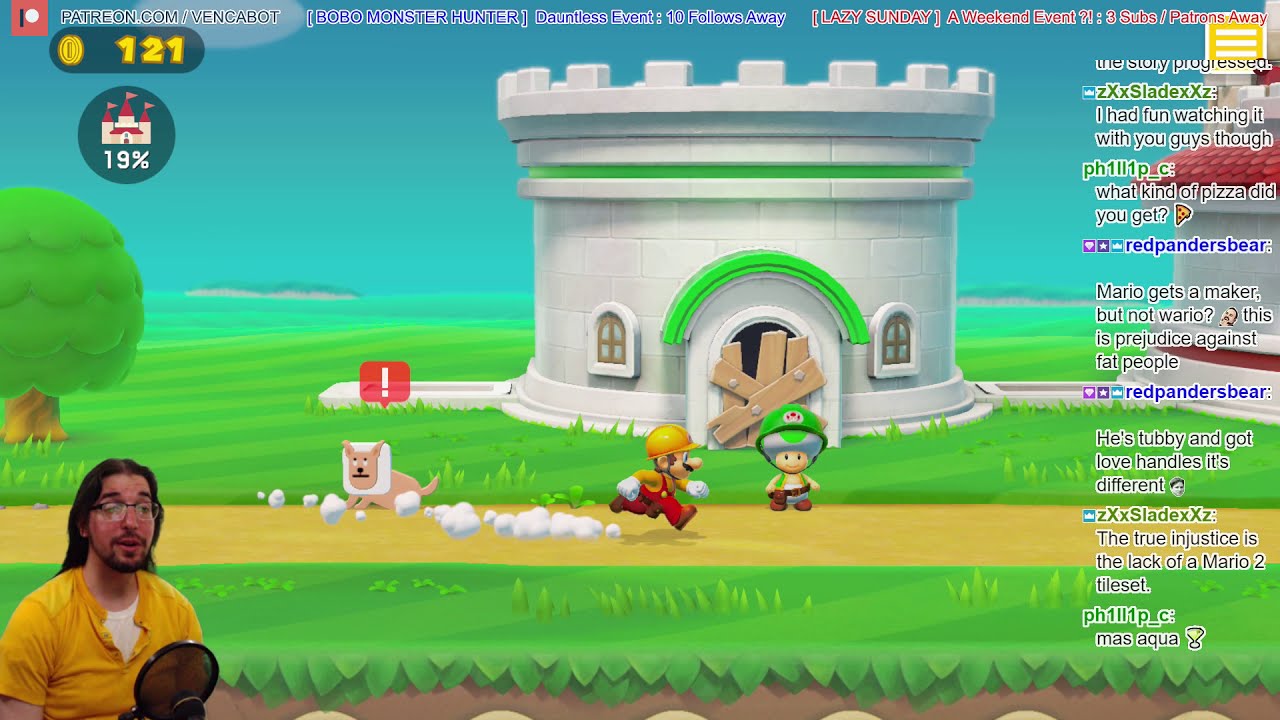The image is a detailed screenshot from a live stream of a Mario game. In the bottom left corner, the streamer, identified as Ben Cabot through his Patreon URL at the top left, is green-screened over the gameplay. He is visible from the chest upwards, wearing a yellow polo shirt with all buttons undone, revealing a thin white cotton undershirt. The streamer has long dark brown hair, glasses with no bottom frame, and a mustache-goatee combo. A microphone peeks into the frame beneath him.

The main game screen shows Mario, dressed in a yellow construction hat and outfit, running to the right past a toad character with a green hard hat in front of a small castle with a boarded-up wooden door. A cat-like creature with a red exclamation mark above its head is also in the scene. The game interface indicates 121 coins and a 19% completion rate at the top left, and the event is labeled "Lazy Sunday" at the top right.

Displayed vertically along the right side is the game chat, with messages such as "I had fun watching it with you guys though," "what kind of pizza did you get 🍕," "Mario gets a maker but not Wario this is prejudice against fat people," and "he's tubby and got love handles it's different." Another chat message reads, "the true injustice is the lack of a Mario 2 tile set."